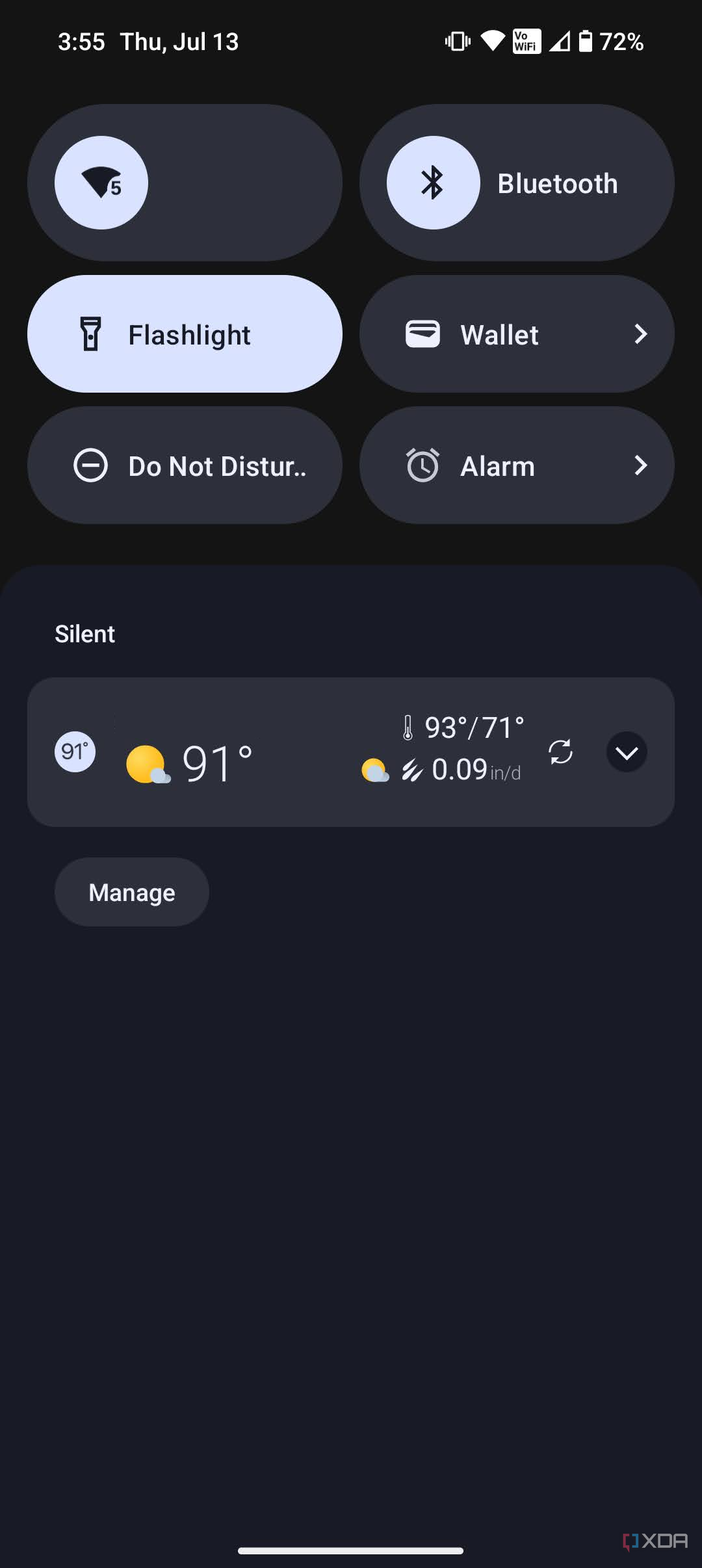A detailed descriptive caption for the image:

---

The image is a screenshot of a smartphone's home screen taken on Thursday, July 13th, at 3:55 PM. At the top left corner, the date and time are displayed, while the top right corner shows several status indicators: 72% battery life, a wireless connection, and the phone set to vibrate mode. Directly below the status indicators, there's a row of quick access icons within cylindrical tabs. The first tab reads "Fly" with the number "5" beside it. Following this, a tab shows the Bluetooth symbol accompanied by the text "Bluetooth."

In the next row, there's a "Flashlight" tab highlighted in white, indicating that the flashlight is turned on. Below this, in a gray tab, is the "Wallet" icon. To the right of the Flashlight tab, another tab displays "Do Not Disturb" with a circle and minus sign symbol. An adjacent tab to the right shows an alarm clock icon labeled "Alarm," accompanied by the text "Silent."

Further down, a weather widget displays the current temperature of 91°F with a sun icon. Next to it, a secondary tab shows the temperature range for the day as 93°-71°F, along with a sun and cloud icon, and "0.09" (possibly indicating precipitation level) with a downward arrow. Below this weather widget, there is a "Manage" option.

Overall, this screenshot captures various functional and informational elements of the smartphone's interface in a detailed and organized manner.